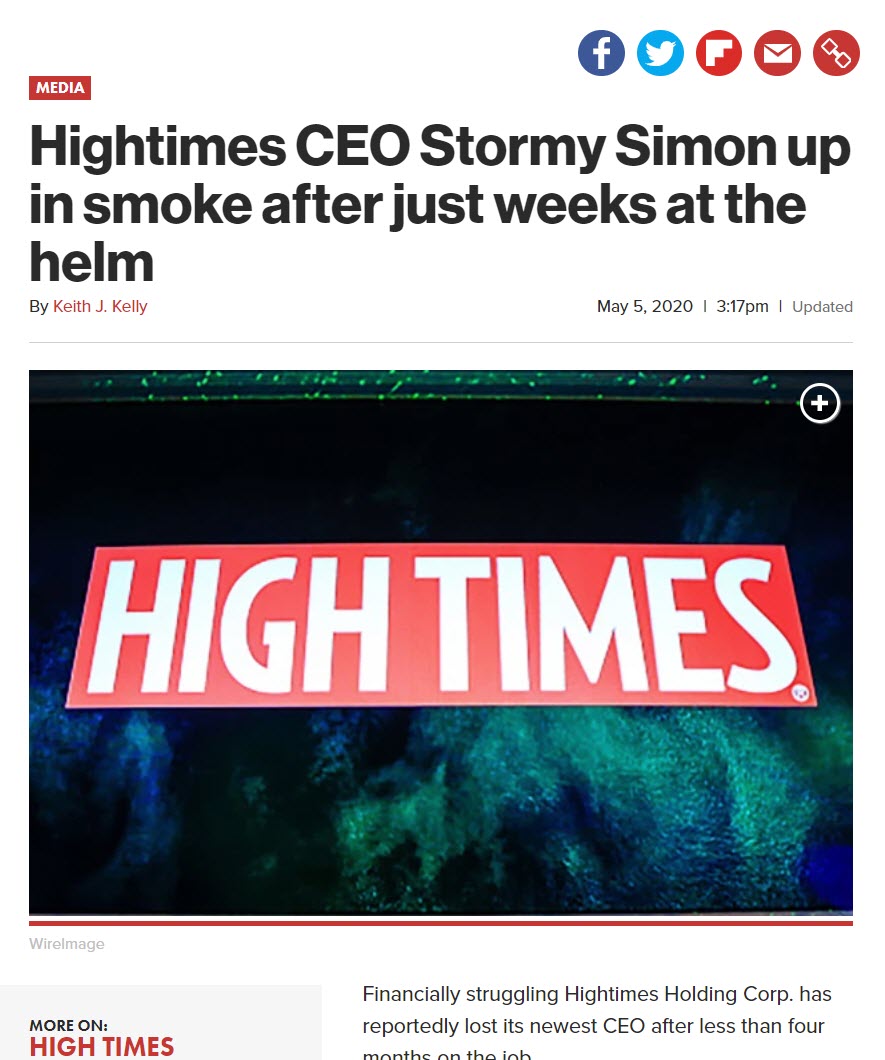The image depicts a news article displayed on a cell phone screen. The image dimensions are taller than they are wide, suggesting it is consistent with a cell phone screen format, though no device is visible. The background is non-existent, blending seamlessly into the black screen.

In the upper right-hand corner, there are five circular icons for social media platforms including Facebook and Twitter. In the top left corner, a red rectangle containing the word "Media" in white font is visible.

The headline reads, "High Times CEO Stormy Simon Up in Smoke After Just Weeks at the Helm" by Keith J. Kelly. The article was published on May 5, 2020, at 3:17 p.m., making it four years old at the time of this caption.

Below the headline, there is an image featuring a "High Times" banner in red with white font against a black background, accompanied by blue and green swirling designs. The body of the article follows underneath this image.

High Times is known as a publication for marijuana enthusiasts, a fact highlighted by the evolving legal landscape of marijuana influencing the industry.